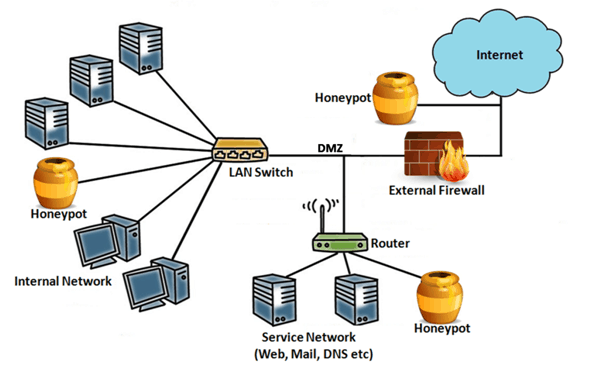This image is a detailed diagram of a computer system setup on a white background. At the top, there are three electronic boxes connected via lines. Below, there is a brown pot with a yellowish band labeled "Honey Pot." Beneath that, it depicts two computers labeled "Internal Network," all lines converging into a box labeled "LAN switch." From there, a line extends to the right, passing through an area labeled "DMZ" and reaching an illustration of a brick wall with flames, labeled "External Firewall," which connects upwards to a blue cloud labeled "Internet." To the left of this setup, another line extends to another "Honey Pot." Further down, a network router is centrally positioned with two boxes below it labeled "Service Network" with annotations such as "Webmail," "DNS," "ETC." These elements interconnect with lines, illustrating the network flow. The diagram includes multiple "Honey Pots," each depicted as gold pots with gold bands, continually emphasizing their integral role in the network.